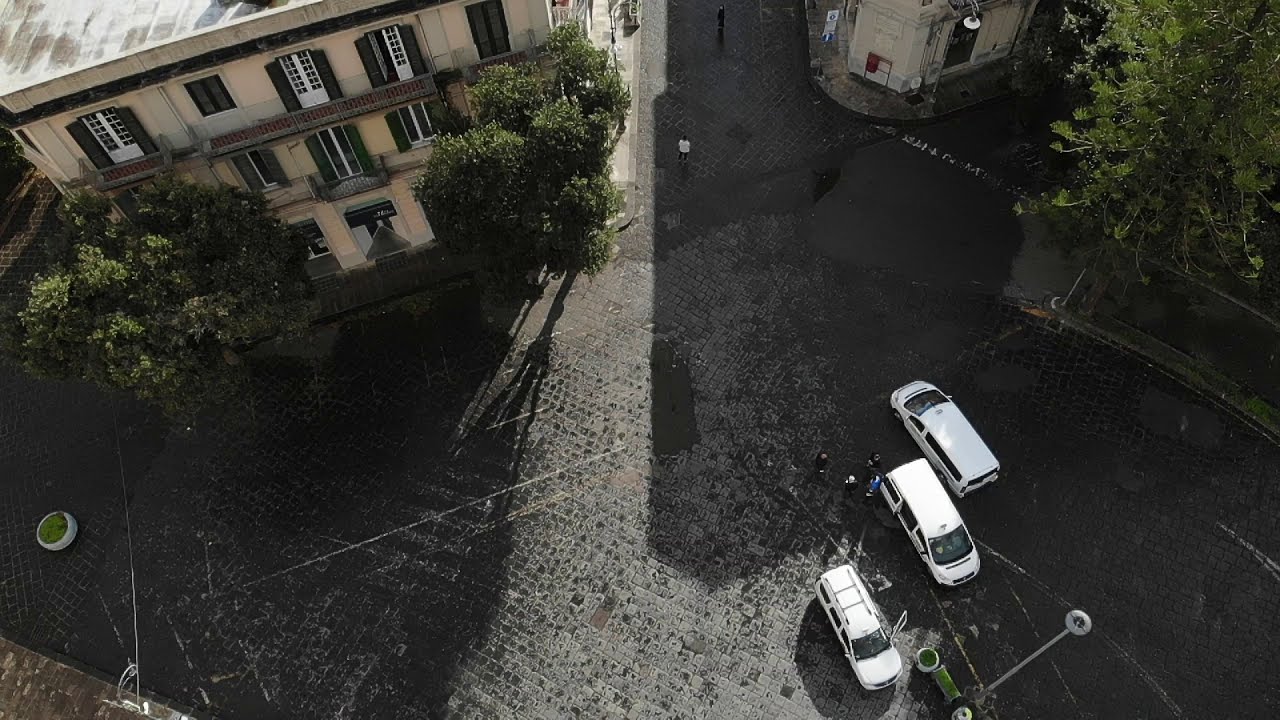This aerial photograph, likely captured by a drone, showcases a well-detailed urban scene with several notable features. The centerpiece is a light pink, three-story building with a flat roof, situated in the top left corner of the image. This building, made of brick, stone, or stucco, displays a mix of black and white windows, surrounded by black trim. To its right and left, tall, bushy green trees create a lush, verdant environment.

Directly beneath the building, three white vehicles, including cars and vans, are parked on a paved, gray surface. Two of these vehicles face downward to the bottom right, while one faces upwards. At the bottom right corner, multiple white plant pots filled with greenery add a touch of nature to the scene.

The image also features numerous roads and sidewalks. There is a roadway extending upward towards the center and another forked road leading off to the top right. The roads, marked with fading white lines, host some pedestrian activity. Additionally, sidewalks run alongside the streets, delineating residential and vehicular areas. A large pine tree is visible at the right side of the forked road, providing further greenery.

The scene is bathed in sunlight, with a distinct strip of light illuminating the center, contrasting with shaded areas cast by buildings to the right. Other buildings, painted in tan or beige hues with darker elements, line the streets, indicating the residential nature of the area. In the background, a white and blue sign is noticeable, hinting at the presence of local amenities. Overall, the photograph captures a bustling residential area, rich in architectural and natural details.